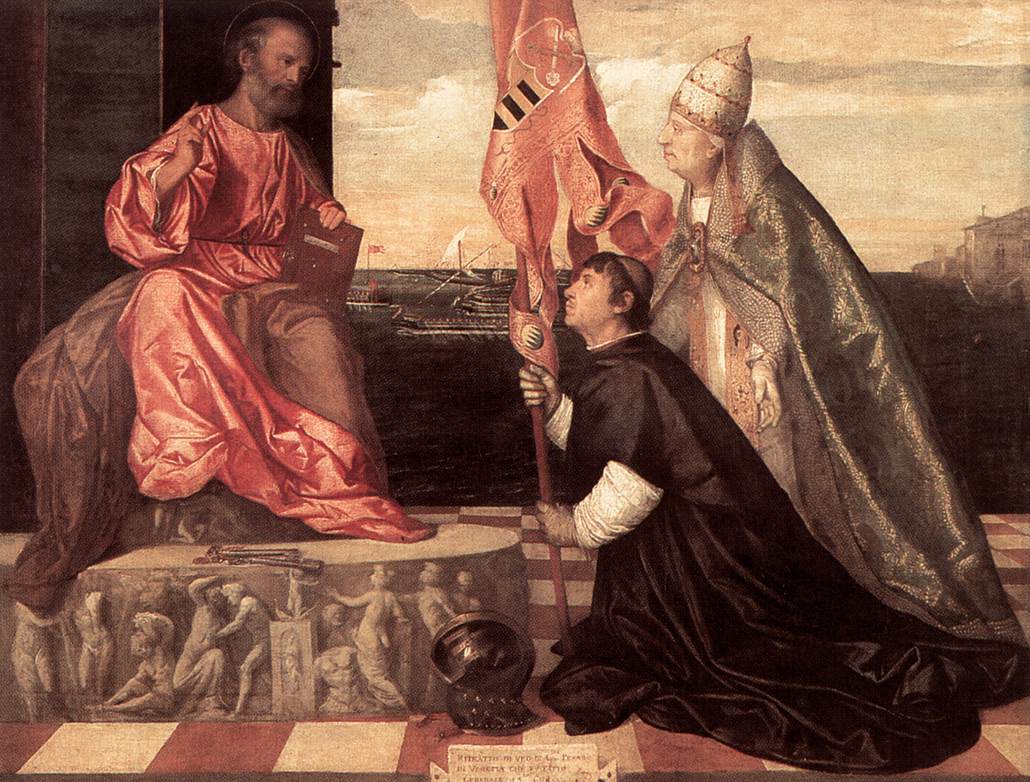The painting depicts a detailed and vivid scene set in the distant past, possibly during the Renaissance or Baroque periods, characterized by muted tones of beige, pink, and silver. On the left side, a distinguished man sits on an intricately carved, grey platform roughly a foot or two off the ground. This man, draped in a light red or hot pink robe that appears slightly too long, revealing its wrinkles, is of older age with sparse, graying hair, a mustache, and brown skin. Holding a book in one hand, he gazes to his right.

In front of this seated man, a younger man in a black robe kneels on green and red square-shaped tiles, holding a flag of an indistinct design, possibly signaling battle. This kneeling figure wears a small cap on his head and possesses striking, white sleeves. Beside him stands an older man, donned in a highly ornate silver gown and a matching tall, crown-like hat. This individual has white hair, hinting at advanced age, and he too looks up at the seated man, conveying a sense of reverence or submission.

In the background, there is a serene body of water with ships floating on it, under a yellowish sky adorned with soft clouds. At the bottom middle of the painting, some text is inscribed, likely in Latin, set against a green background. A black helmet lies on the ground, adding to the historical and possibly military context of the scene.